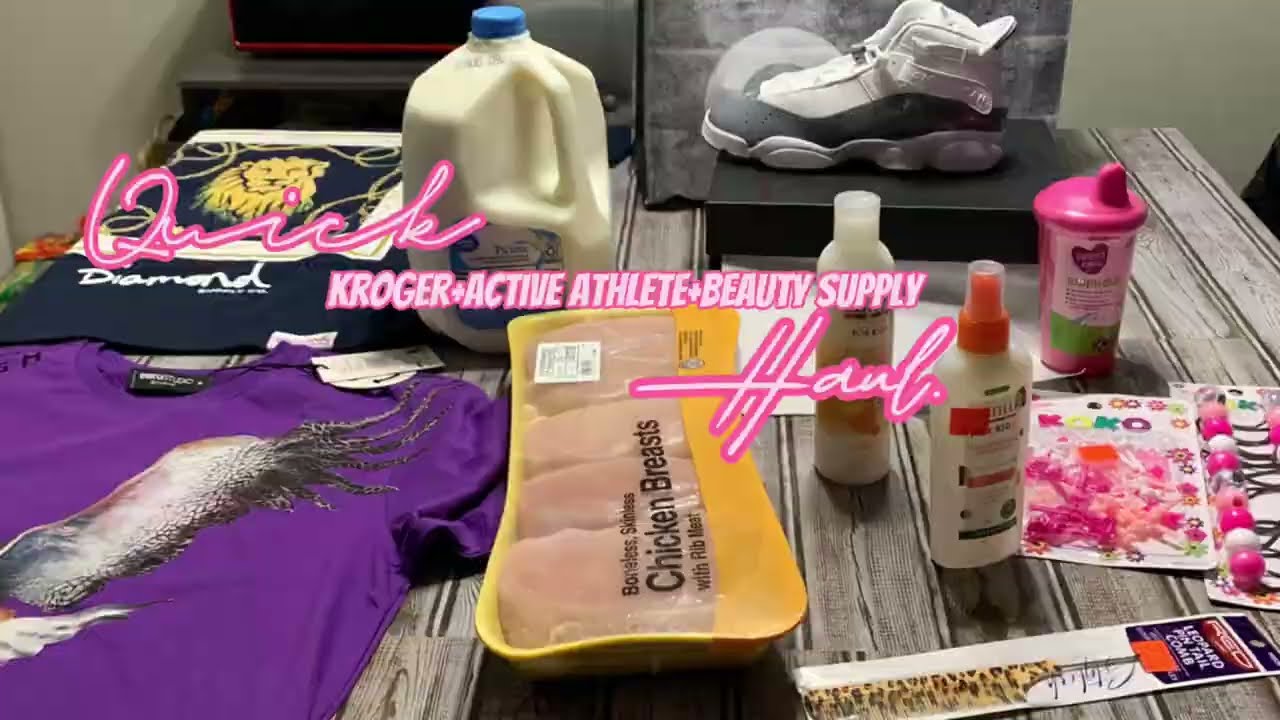On a gray wooden table, there is a diverse assortment of items scattered around a vibrant central banner. The banner prominently features the words "Quick Kroger Plus Active Athlete Plus Beauty Supply Haul" written in white cursive outlined in pink. Surrounding this banner are numerous distinct items. 

In the center bottom, there's a family-sized tray of boneless, skinless chicken breasts wrapped in yellow paper. To the left, a purple t-shirt with a white wing design lies next to a drawing of a lion’s head with the word "Diamond" in white print on a black background. Above that is a package of crafting supplies including pigtail holders and hairbands colored pink and white.

To the right, a gallon of milk with a blue lid stands tall. Nearby, a toddler's pink-topped sippy cup sits next to two bottles of hair products and a leopard print comb. In the upper right corner, a high-topped, black-and-white tennis shoe is displayed on top of a shoebox, encased in a glass box. This eclectic variety of groceries, apparel, and beauty supplies reflects a quick yet diverse shopping haul, creatively showcased in the image.